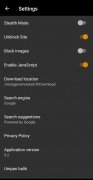This image is a screenshot of a cell phone screen. At the very top, there is a black header bar with a white left-pointing arrow. Next to the arrow, partially blurred white text appears to begin with the letters "B" and "E". 

The rest of the image is set against a dark grey background and is significantly blurred. On the left side of the screen, there are approximately ten rows of short, white text entries, though the text is unreadable due to the blurriness. Some of these rows have smaller text beneath them, but it is also illegible.

To the right of these rows of text, there are toggle switches for each row. The first row features a toggle switch in the "off" position, indicated by a white circle on the left with a grey bar extending to the right. The second row presents a toggle switch in the "on" position, marked by an orange circle on the right with a lighter orange bar extending to the left. The pattern continues with the third row showing an "off" switch and the fourth row an "on" switch, and so on.